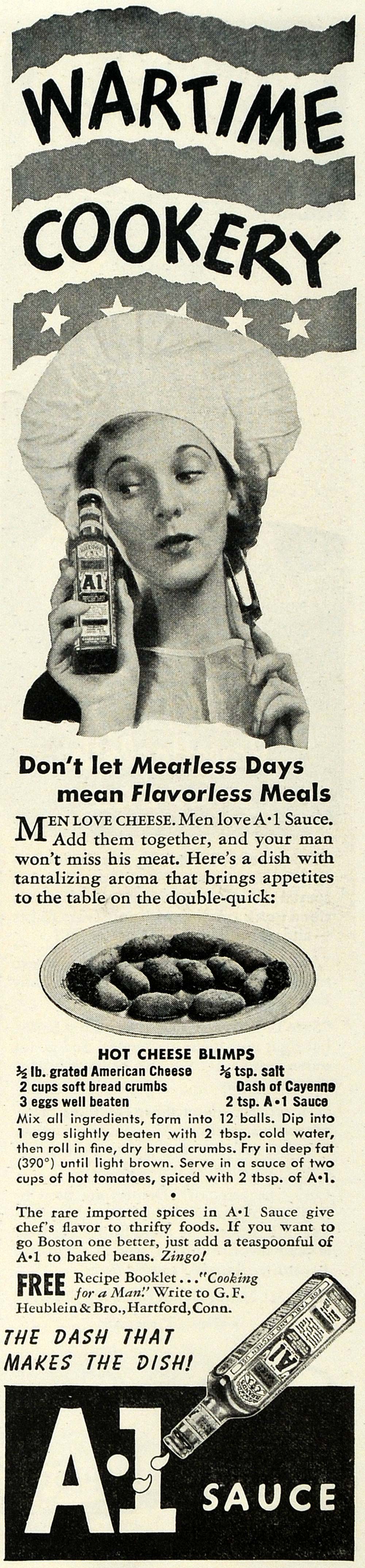This black-and-white World War II-era advertisement for A1 sauce, likely from a newspaper, exudes nostalgia with its slightly cream-tinted monochrome palette. Dominating the top section, the bold text reads "Wartime Cookery," adorned with patriotic stripes and stars, underscoring the context of rationing during the war years. Centered below this heading is an image of a woman wearing a traditional chef's hat, holding a bottle of A1 sauce in one hand and a two-pronged kitchen fork in the other, promoting the sauce as a solution to flavorless, meatless meals. She stands as a symbol of home-front ingenuity, countering the scarcity of meat with culinary creativity. Accompanying the image, the text emphasizes, "Don't let meatless days mean flavorless meals. Men love cheese, men love A1 sauce. Add them together and your man won't miss his meat." Further down, a tantalizing description promises a dish with an irresistible aroma: Hot Cheese Blimps, designed to bring appetites to the table quickly. The lower section features a clear picture of the A1 sauce bottle alongside its logo, completing the advertisement with the critical message that A1 sauce can transform even the simplest dishes into something special.